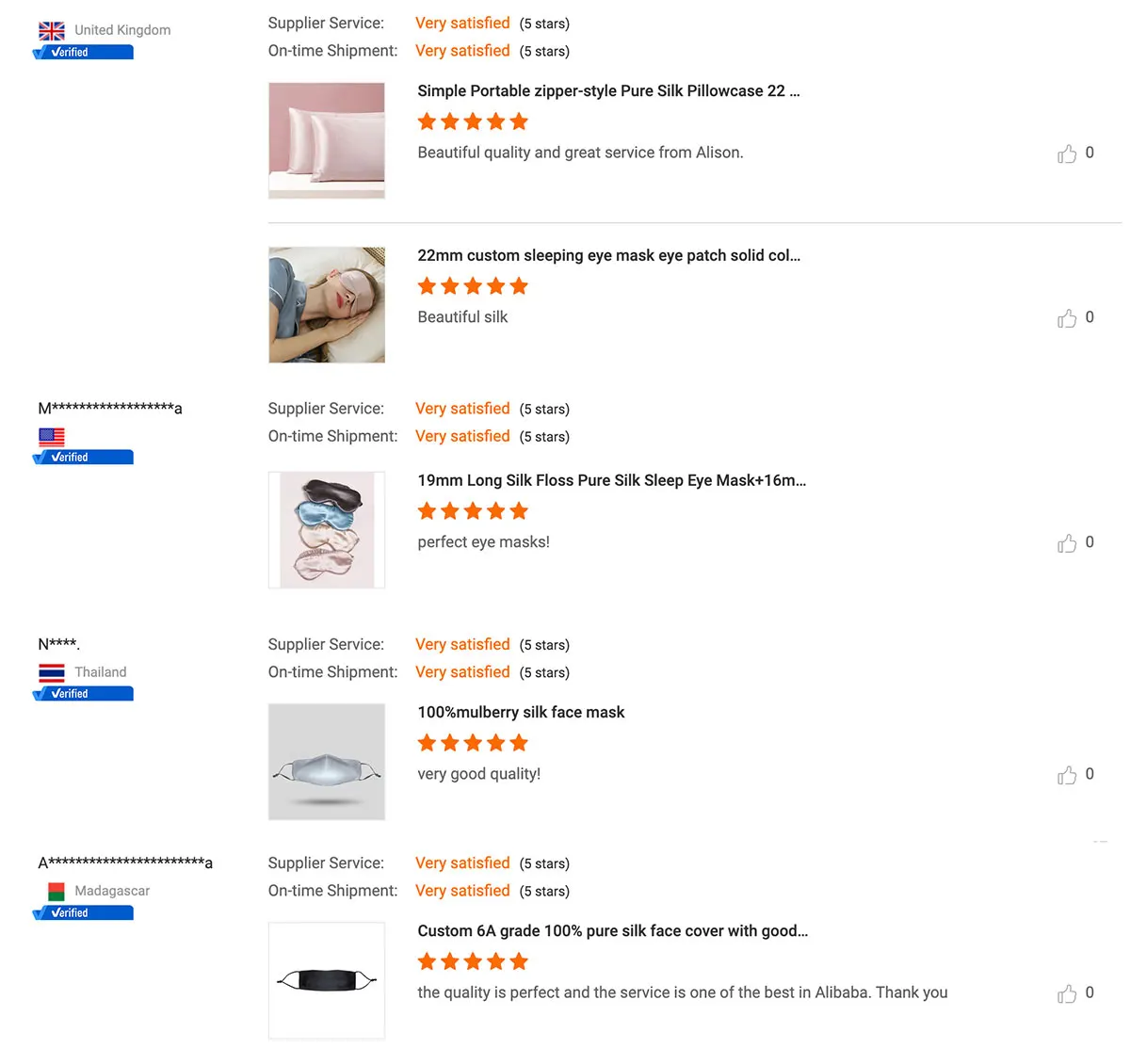This image displays a collage of customer reviews and ratings for various silk products. It features detailed feedback on supply service, on-time shipment, and product satisfaction levels. 

1. **Reviewer from the United Kingdom**: 
   - Product: 22mm custom sleeping eye mask 
   - Rating: ★★★★★ 
   - Review: "Beautiful quality and great service from Allison."

2. **Reviewer from the United States**: 
   - Product: Sleeping eye mask 
   - Rating: ★★★★★ 
   - Review: "Simple, portable style, made from pure silk. Very satisfied."

3. **Reviewer from Thailand**: 
   - Product: Pure silk eye mask and face mask 
   - Rating: ★★★★★ 
   - Review: "Exceptional quality of 6A pure silk, perfect fit, and impeccable service."

4. **Reviewer from Madagascar**: 
   - Product: Custom 6A silk face mask 
   - Rating: ★★★★★ 
   - Review: "Multiple colors available, superb quality, and outstanding service."

All reviews convey a sense of high satisfaction with Alibaba's products and services, underlining the excellent craftsmanship and delivery reliability.